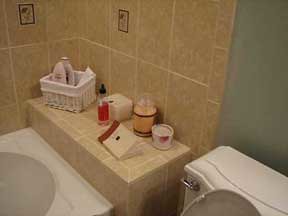This photograph showcases a modern bathroom with a stylish design. The walls are adorned with wide, large tiles that feature integrated images and designs, giving the space a contemporary yet elegant appearance. The light-colored grout provides a subtle contrast, enhancing the overall look of the tiles. A shelf, crafted from the same tile material, extends along the wall, blending seamlessly with the decor.

Despite its vintage appearance, the toilet tank is a high-end, late model designed to mimic a classic style, as indicated by its modern handle. The quality and craftsmanship extend to the bathtub, which is expertly installed with nearly invisible caulking, emphasizing the meticulous attention to detail in this bathroom.

On the built-in shelf next to the tub, various items are neatly arranged. These include a book, a candle or fragrance device, a dispenser containing oil or lotion, a tissue box, and a small light-colored wicker basket. The basket holds an assortment of personal care products, such as powder or shampoo and a tube of cream. The light tan and light brown tile graphic serves as a tasteful backdrop to these accessories, completing the tranquil and inviting atmosphere of the bathroom.